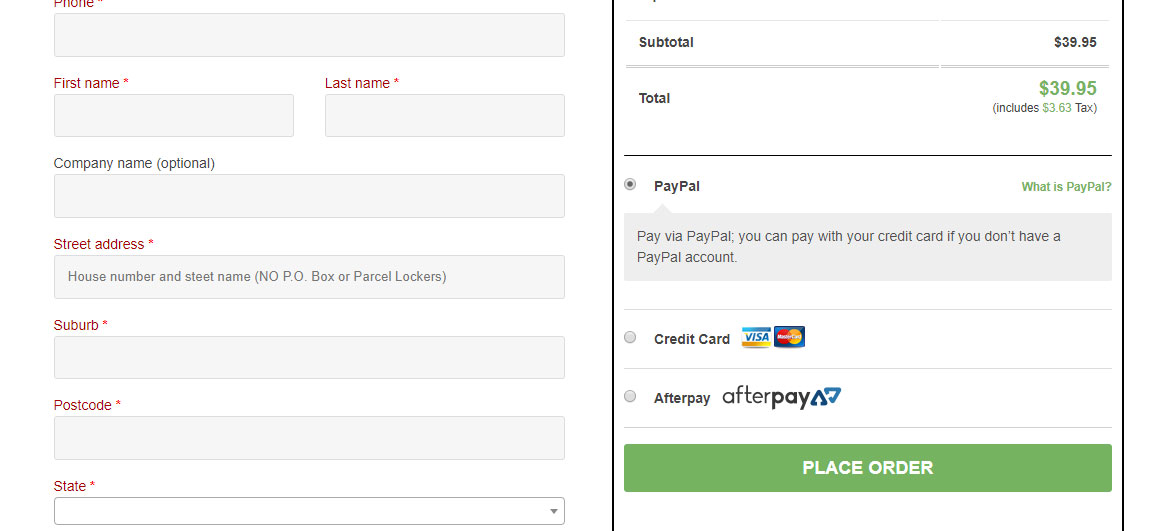**Descriptive Caption:**

On a white background, the image showcases a structured user input form. Starting from the top left, the heading reads "Phone" with a gray rectangular text input box positioned immediately below it. Following this is a "First Name" label, accompanied by a gray text area beneath. Adjacent to it on the right side, the label "Last Name" appears, also with a corresponding gray text area below.

Continuing down, the form displays "Company Name" with "(optional)" in parentheses, and a text box for input underneath. Directly below this, the field labeled "Street Address" is shown with a text box designated for entering the house number and street name. Next to this, parentheses specify, "No PO Box or parcel lockers."

Further down the form, the labels proceed with "Suburb" followed by a text box, "Postcode" with its own text box, and finally, "State," which is paired with a drop-down menu for selection. The vertical layout is flanked by two thin black lines running vertically on the left and right sides of the image.

At the top, a light gray horizontal line demarcates the boundary, with the subtotal amount "Subtotal: $39.95" displayed beneath it. This is followed by another light gray horizontal line that runs across the width of the image. The overall design ensures clarity and ease of navigation for user input.